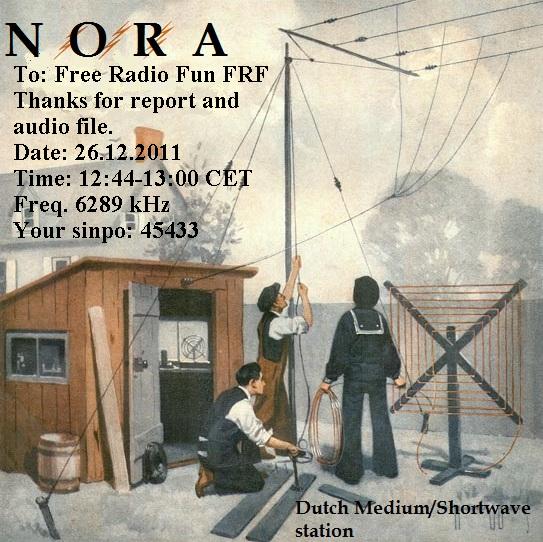The hand-drawn advertisement for a radio station features three men dressed in late 1800s attire, comprising overalls, jumpsuits, vests, and old-style hats, setting up an intricate radio tower with multiple wires. One man is gripping electrical wiring, another kneels on the ground holding a rod connected to the cable, and the third holds a coil of orange wire, which is wrapped around an antenna to the right. Behind them stands a small wooden shack with an open door, a wooden barrel, and a wooden plank. The top left corner of the image contains the text: "NORA to Free Radio Fun FRF. Thanks for report and audio file. Date: 26-12-2011, Time: 12-44-1300 CET, Frequency: 6289 kHz, Your Simpo S5-45433." In the bottom right corner, it reads: "Dutch Medium Shortwave Station."